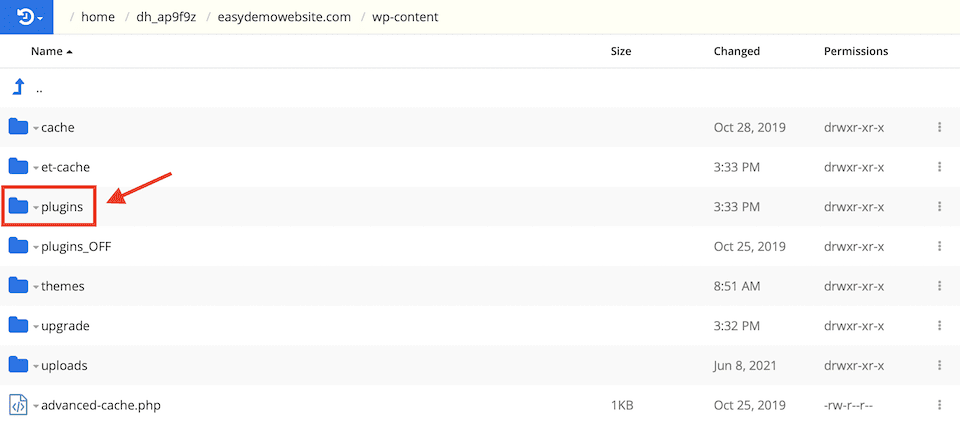A detailed screenshot of a computer screen displaying a file directory. The interface reveals a table with predominantly white rows, interspersed with very pale grey alternating rows. Located at the top left of the image is an icon—a partially complete circle arrow rotating counterclockwise against a blue background. Adjacent to this icon is a breadcrumb trail that reads: "home > dhap9f9z > easydemowebsite.com > wp-content."

Beneath this, the table has four headings: "Name," "Size," "Changed," and "Permissions." Directly under these headings, the first row features an up arrow in blue, indicating a return to the previous directory level. Following this are seven rows, each marked with a blue folder icon symbolizing different directory folders. The details are as follows:

1. **cache** - Last modified on October 28, 2019, with permissions set to `drwxr-xr-x` and featuring a three dots icon on the far right for more options.
2. **et-cache** - Last modified at 3:33 PM, with identical permissions `drwxr-xr-x`.
3. **plugins** - This row is emphasized with a large red rectangle and a red arrow pointing towards it. It was last modified at 3:33 PM with the same permissions `drwxr-xr-x`.
4. **PLUGINS-OFF** (in capitals) - Last modified on October 21, 2019.
5. **themes** - Last modified at 8:51 AM.
6. **upgrade** - Last modified at 3:32 PM.
7. **uploads** - Last modified on June 8, 2021.

The last row of the table showcases a file named **advanced-cache.php**. This file is 1 kilobyte in size, last modified on October 25, 2019, and has permissions set to `-rw-r--r--`.